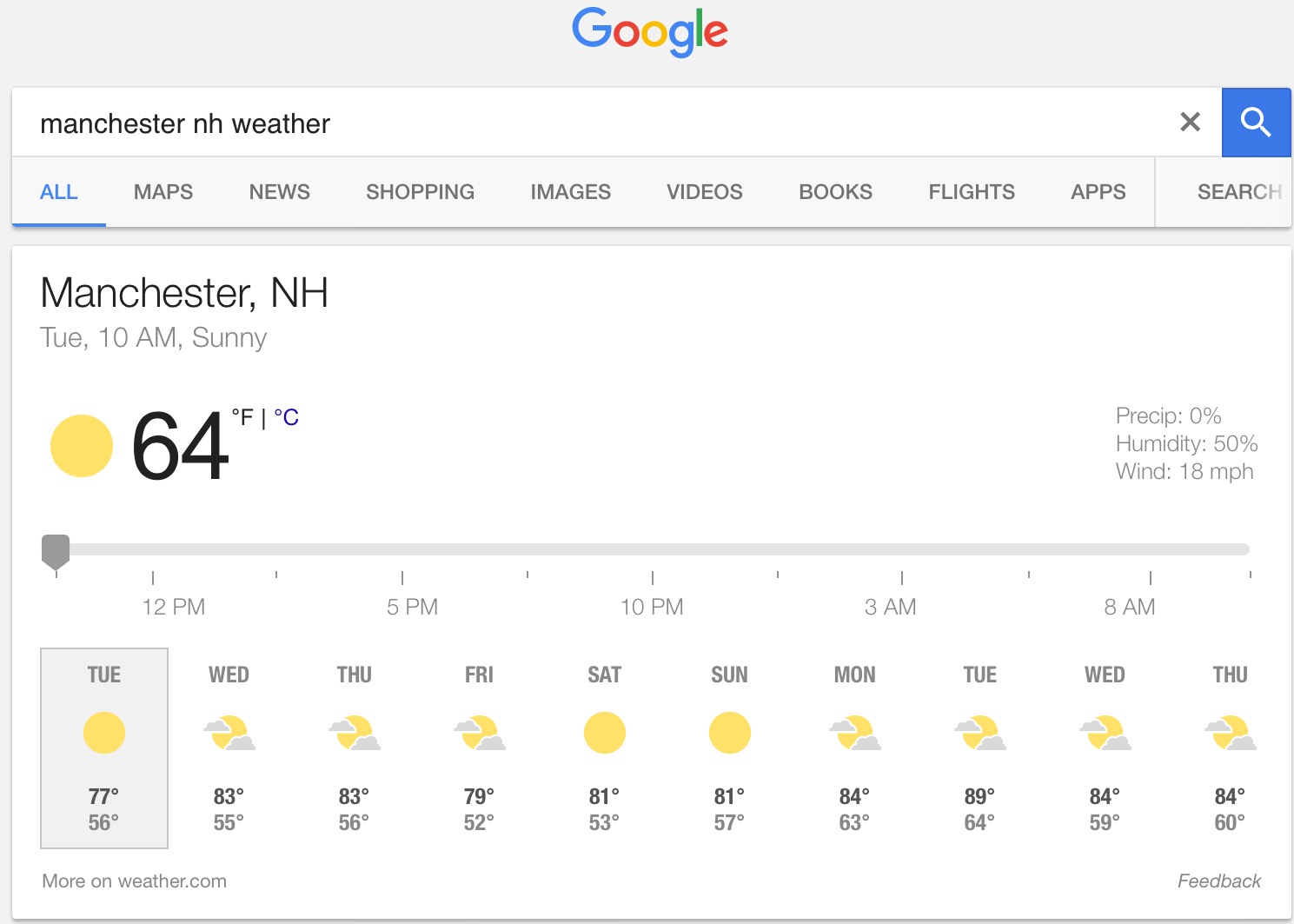The image features a classic Google search homepage layout on a grey background. Prominently displayed at the center is the word "Google," rendered in its iconic multi-color scheme: blue, red, yellow, blue, green, and red. Below the logo is a white search bar, within which are the black query terms "Manchester, NH weather." To the right of the search bar is a grey 'X' icon and a blue search button with a white magnifying glass.

Beneath the search bar, a horizontal navigation menu features several categories: "All" in blue and underlined, followed by "Maps," "News," "Shopping," "Images," "Videos," "Books," "Flights," "Apps," and "More," all rendered in grey.

The main body below this menu displays weather information for Manchester, New Hampshire. The current condition indicates 2:10 AM and sunny, represented by a yellow sun icon. The temperature is shown as 64°F (18°C). Additionally, there are detailed meteorological data: precipitation at 0%, humidity at 50%, and wind speed at 18 MPH. 

A bar graph beneath this information forecasts temperatures at various times—12 PM, 5 PM, 10 PM, 3 AM, and 8 AM—though it's noted this feature may not be current Google practice.

At the bottom, a blue circle highlights the day "Tuesday," accompanied by a sun icon and temperatures 77°F/56°F. The forecast extends for the next week, detailing daily highs and lows, with the highest predicted temperature at 89°F and the lowest at 52°F.

This descriptive caption thoroughly encapsulates the visual details and textual information displayed in the image of the Google search result for Manchester, NH weather.